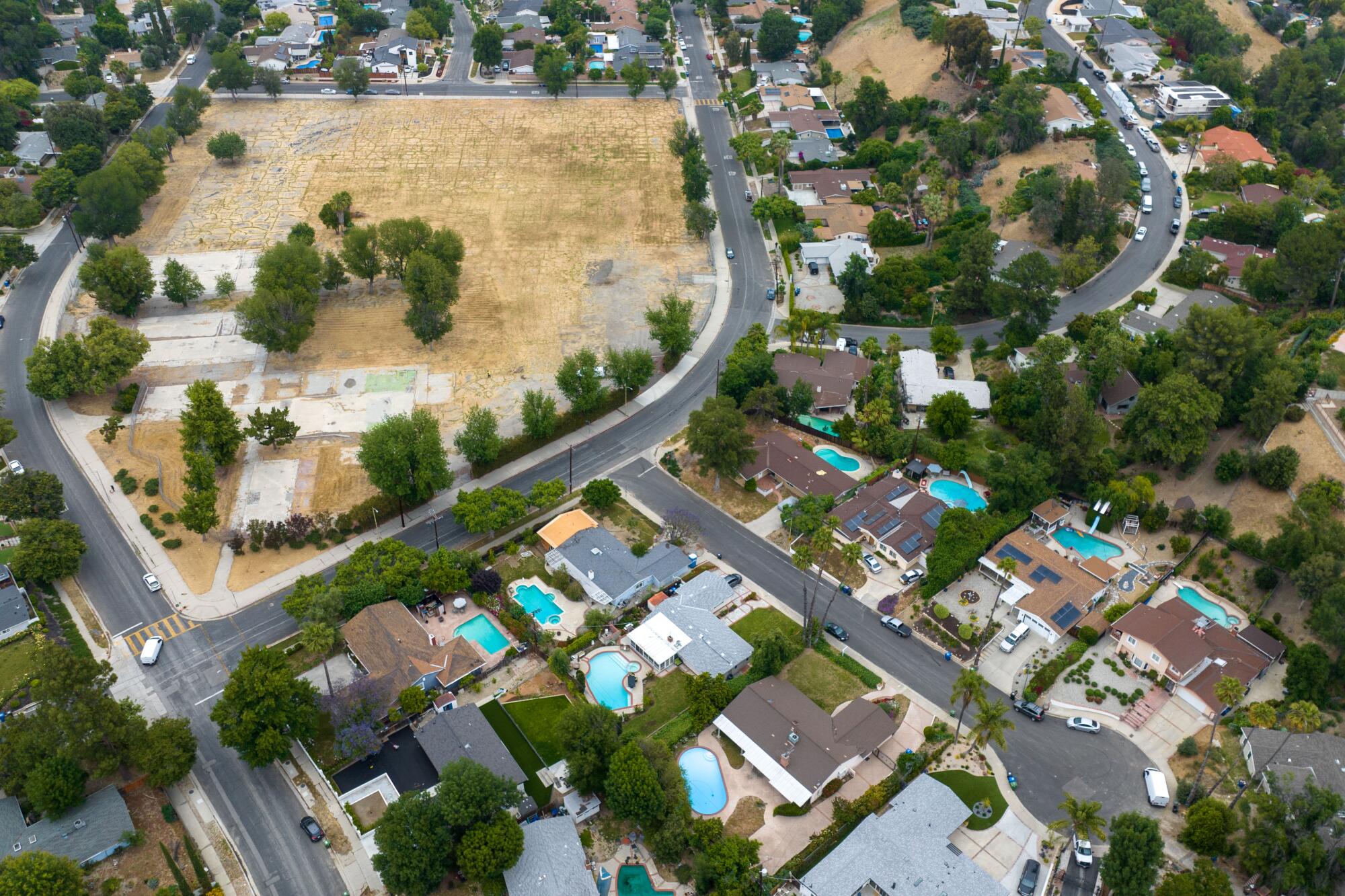This detailed aerial photograph provides a comprehensive view of a suburban neighborhood. In the foreground, the image showcases a row of houses lining a street, each featuring swimming pools in their backyards. These pools stand out distinctly with their turquoise blue color, and you can count about nine of them quite clearly. Many other houses throughout the neighborhood also have pools, dotted among the various residences.

The neighborhood is enriched with lush, green deciduous trees that fill the spaces between houses, roads, and yards, contributing to a serene suburban feel. Numerous quiet streets and intersections wrap around the properties, creating a network that includes cul-de-sacs with parked cars. 

Towards the upper left of the image, there is a large empty field dotted with trees and scattered concrete slabs, likely designated for future housing development. This area contrasts with the more densely packed sections of the community. 

In the center of the neighborhood, the photograph reveals fields that may be designated for recreational use, possibly park or sports fields, and slight hills that add some terrain variation to the otherwise predominantly flat land. 

To the right of the image, there are more trees and additional houses that align with the road, creating a densely wooded section of the neighborhood. Overall, the image captures a well-planned and verdant residential area, characterized by its ample greenery, numerous pools, and extensive housing.